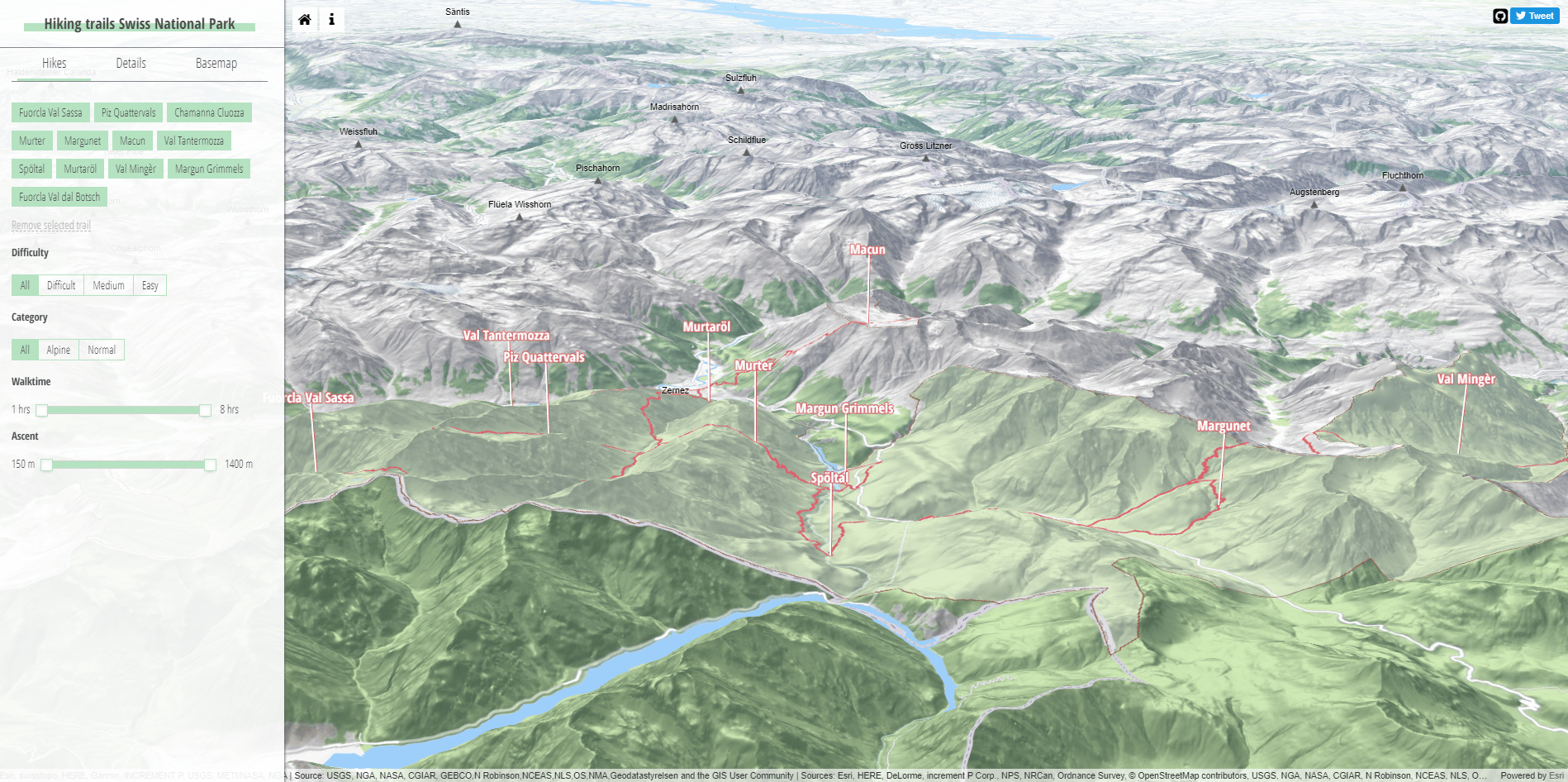This image is a detailed, computer-rendered topographical map of the Swiss National Park, showcasing hiking trails and landscape features. The primary color scheme includes muted greens to indicate vegetated areas, grays for mountainous terrains, and blues for bodies of water. At the top left corner, the image is labeled "Hiking Trails, Swiss National Park" along with additional trail details. 

Prominent on the map are orange and red lines representing hiking trails, clearly marked with names such as Morgan, Graham, Murier, Spada, and Margonet, indicating their routes through different park areas. Specific trails' difficulties and other relevant information are detailed on the left-hand side.

In the bottom left, a long blue river, part of the area's drainage system, cuts through the lowest elevations. The park's landscape transitions from green vegetated areas in the foreground to predominantly gray, vegetation-free mountainous regions in the middle and background. As the map extends further, a tiny, blue sky sliver is visible, adding depth to the illustration.